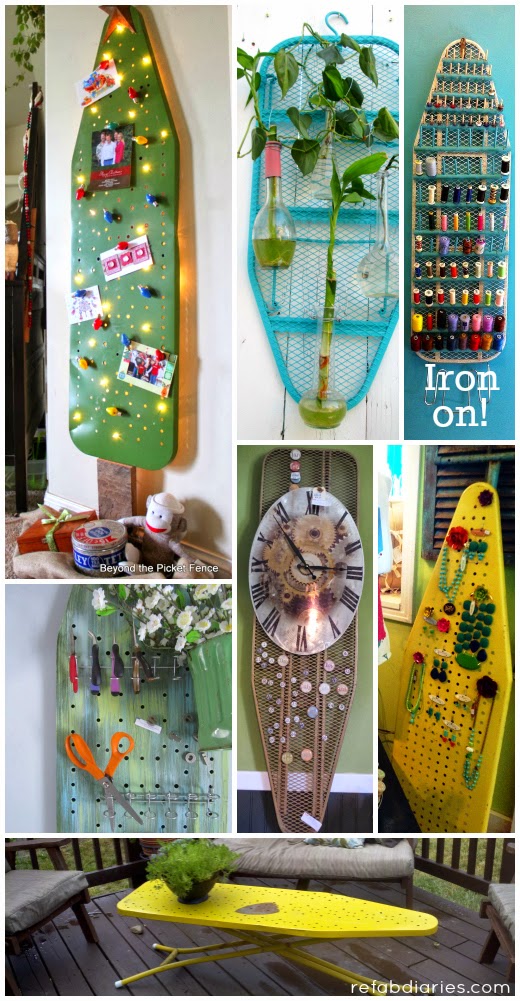This tall rectangular image, sourced from refabdiaries.com, showcases an array of inventive crafts made from repurposed ironing boards. At the upper left, an ironing board turned Christmas tree is adorned with a green cover, retro Christmas bulbs, family photos, and a wooden stem, enhanced with backlit ornaments. A stuffed monkey and presents, including an orange-wrapped gift, complete the festive display. Adjacent, an outdoor wall-mounted ironing board features an array of potted plants. Beneath it, another board serves as an organizer for spools of thread with added shelves. The bottom-most board, painted bright yellow, functions as a vibrant plant stand.

Central to the display, a brown ironing board takes on the appearance of a grandfather clock, complete with a centrally placed clock and coin decorations. Flanking it, the leftboard uses wire hooks to hang various items including flowers, threads, and scissors, while the rightboard, also yellow, utilizes its holes to neatly hang colorful jewelry.